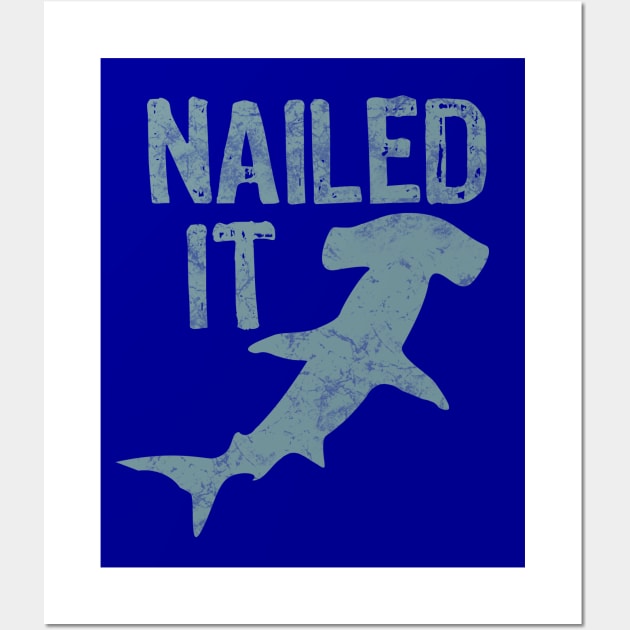This image depicts a vibrant, computer-generated poster set against a thick white border on a grayish white surface. The main body of the poster showcases a deep, dark blue background with a sponge-textured, painted effect. Dominating the upper portion in large, weathered, all-caps lettering is the phrase "NAILED IT," rendered in a light blue, almost white hue that appears stamped or sponged on. Beneath the text, a substantial silhouette of a hammerhead shark stretches across the majority of the poster, painted in the same bluish-white color. The shark is purely an outline without intricate details, reinforcing the simplistic yet striking aesthetic of the design. This piece of decorative art, devoid of any watermarks, seems to celebrate or commemorate an event, such as a successful fishing trip, making it a fitting addition to a wall display.